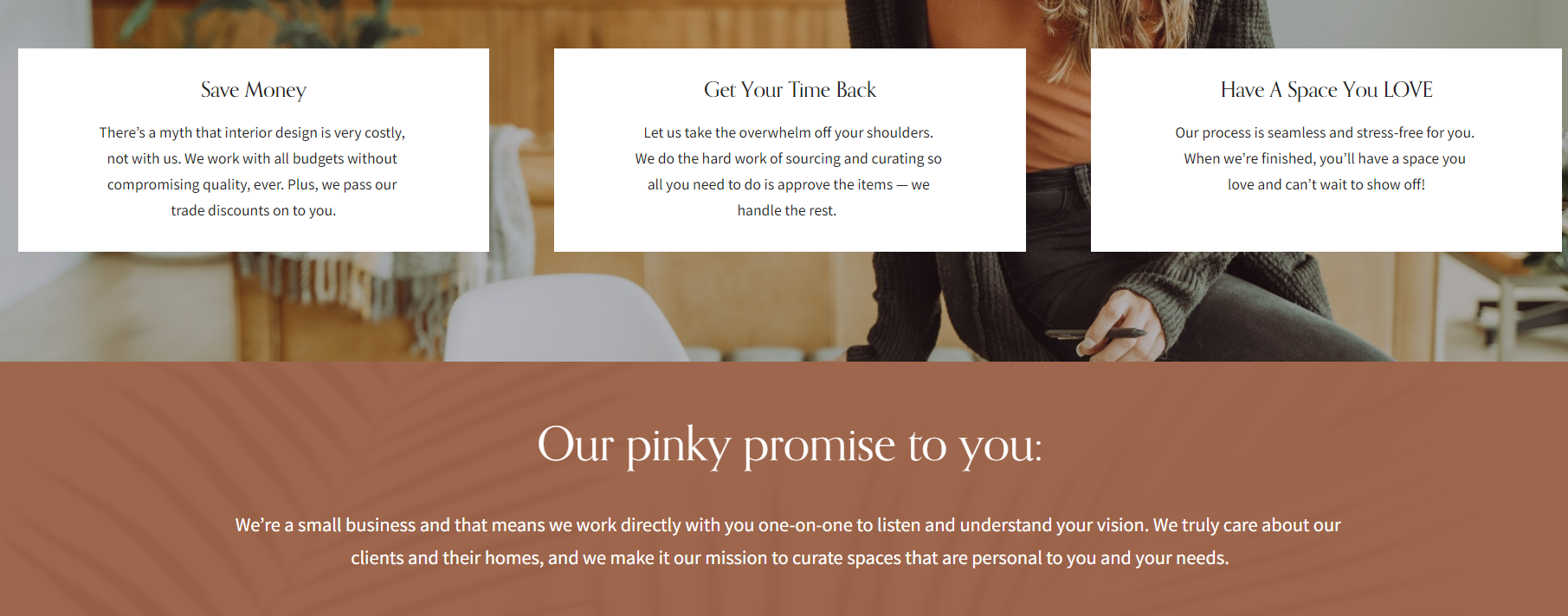The image features three white square boxes with black text, set against the backdrop of an interior room. Each box contains a message highlighting different benefits of the interior design service:

- The box on the left states, "Save Money: Interior design can be costly, but not with us. We work with all budgets without compromising quality, and we pass our trade discounts on to you."
- The middle box reads, "Get Your Time Back: Let us take the overwhelm off your shoulders. We handle the hard work of sourcing and curating items, so all you need to do is approve the selections while we manage the rest."
- The box on the right says, "Have a Space You Love: Our process is seamless and stress-free. When we're finished, you'll have a space you love and can't wait to show off."

The background showcases an inviting room. In the foreground, a person sits atop a table surrounded by white chairs. They are dressed in a black jersey, a brown t-shirt, and black trousers.

At the bottom of the image, white text on a brown background declares a message from the business: "Our pinky promise to you: As a small business, we work directly with you one-on-one to listen and understand your vision. We truly care about our clients and their homes, making it our mission to create spaces that are personal to you and your needs."